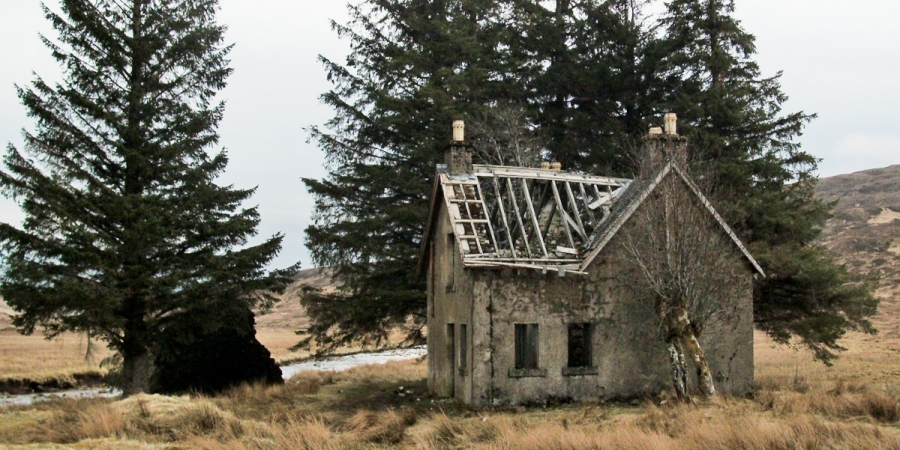This image depicts a dilapidated, two-story house situated in an arid, dry grassland. The house's once sturdy structure is now marred by significant fire damage, with its blackened, collapsed roof revealing the skeletal framing and open, pane-less windows that gape into the empty interior. Visible in the house's layout are several chimney stacks, further highlighting its aged and forsaken state. Directly behind the house stand three towering evergreens, their tops cut off from view, among which are wilted, leafless trees that add to the scene's somber atmosphere. A small stream flows beyond the house, meandering through the desolate landscape. The sky overhead is a light, nearly washed-out blue, hinting at a clear but stark day. To the right of the house, there is a small hill, with no other signs of civilization in sight. The overall scene captures the eerie beauty of abandoned and forgotten places, emphasized by the contrast between the natural landscape and the decaying human structure.